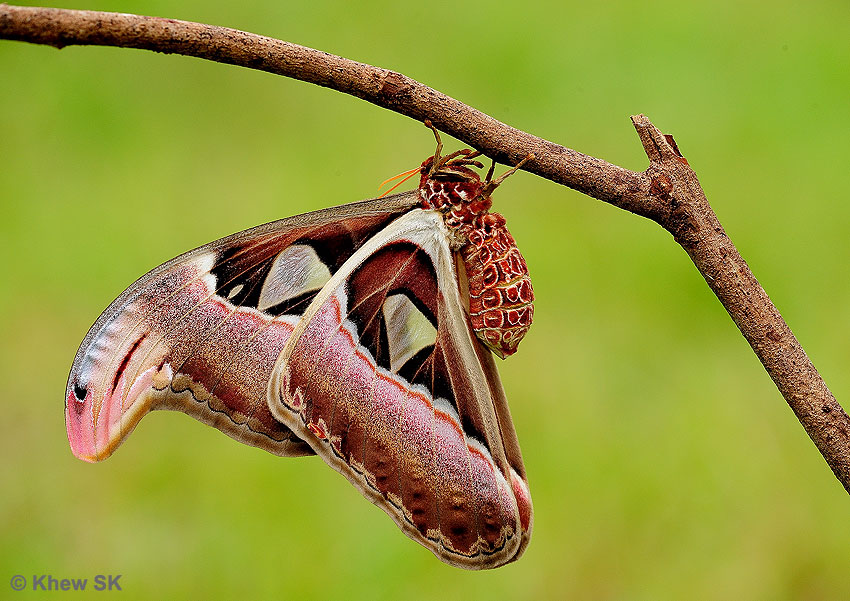The professionally taken nature photograph showcases a detailed close-up of a butterfly resting on a tree branch. The photo is copyrighted with "KHEW S K" in the lower-left corner. The background features a beautifully blurred blend of greens and yellows, spotlighting the intricately detailed scene in the foreground. The brown tree branch, appearing almost diagonally, is richly depicted with visible knots, where the bark has been scraped off.

The main subject, a uniquely patterned butterfly, clings delicately to the branch. Its body is a sublime mix of red and white, adorned with small white dots. The insect’s legs and fuzzy body are rendered in stunning detail. It boasts two prominent orange antennae. Its wings, fabulously spread, are a captivating combination of pink, white, brown, black, and maroon. The inner wings feature a striking white diamond shape encircled by red, while the outer wings have a soft, dusty look. The meticulously captured image allows for an appreciation of the butterfly's vibrant colors and textures against the blurred green backdrop.